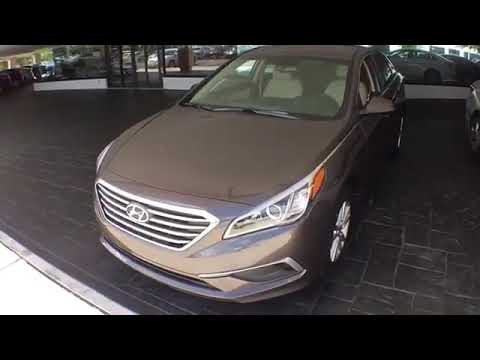The image depicts a bronze or taupe-colored SUV parked inside a parking garage, identifiable as a Honda by the "H" on the front grill. The interior features pale white or beige seat covers and headrests, indicating a light-colored upholstery. The garage floor is composed of dark gray rectangular tiles. In the background, other parked cars are visible, along with a view extending to the surrounding neighborhood outside.